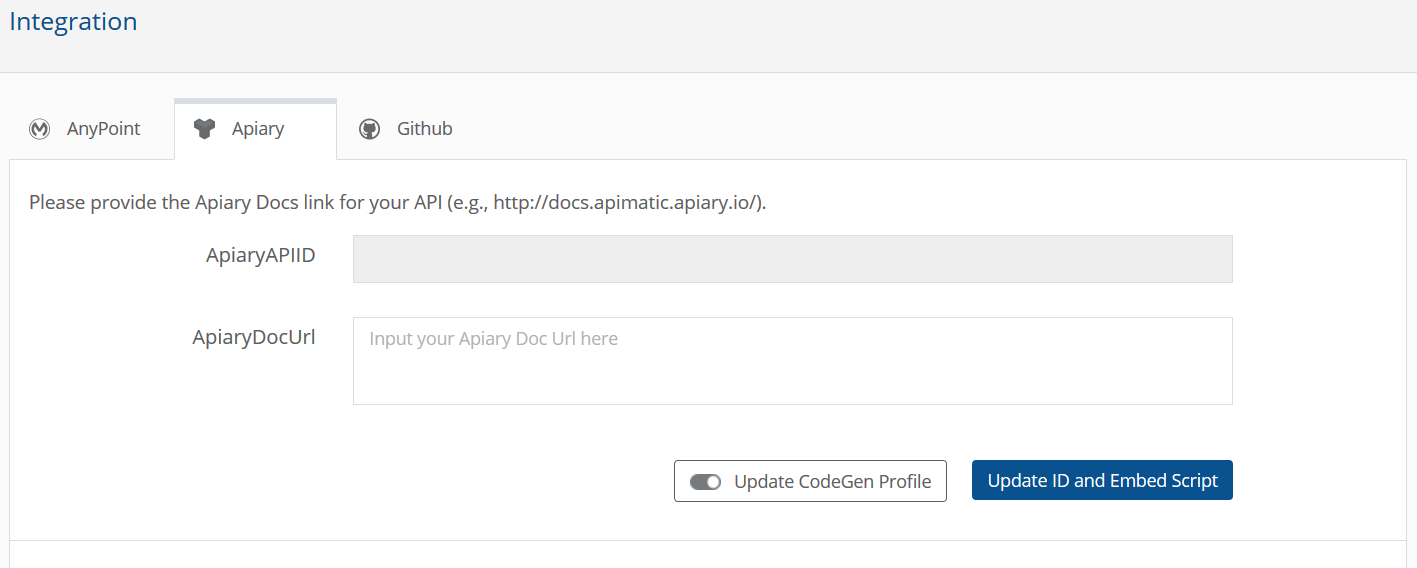The image depicts a user interface on a website, specifically a section requiring user input within a form field. At the top left corner, the heading "Integration" is clearly visible. Directly below this, several options are listed, such as "AnyPoint," "Parry," and "GitHub." The "Parry" tab is currently active and displayed on the screen. This tab contains the instruction: "Please provide the Parry or Parry Docs link for your API." Following this directive, there is a parenthetical reference linking to an example website for further guidance. Below the instructions, an empty input field is present, prompting the user to enter the specified ID or URL related to their API documentation.